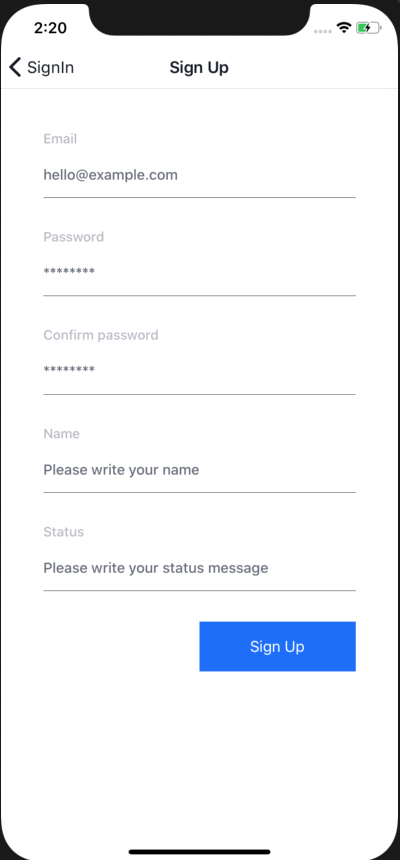The image is of a cell phone displaying a "Sign Up" screen. In the background, the device status indicators are visible: the top left corner shows "2:20" in black, while the top right corner displays the Wi-Fi signal and a battery icon that is currently charging and approximately 50% full. 

On the screen, the interface is primarily text-based with input fields delineated by light gray lines. On the left-hand side, there is a black left arrow followed by the text "Sign In." Centered at the top of the screen, "Sign Up" is prominently displayed. 

The first input field below the gray line is labeled "Email," with a placeholder text "hello@example.com." Below this, another gray line separates the next field, labeled "Password," which is followed by a series of dots or asterisks to represent hidden characters. Another gray line separates the "Confirm Password" field, which has the same dot or asterisk representation for the input. 

Further down, another gray line precedes the "Name" field, with the placeholder text "Please write your name." Below this, yet another gray line delineates the "Status" field with the placeholder text "Please write your status message."

At the bottom right of the screen, there is a prominent blue rectangle button with "Sign Up" written in white, centered within the button.